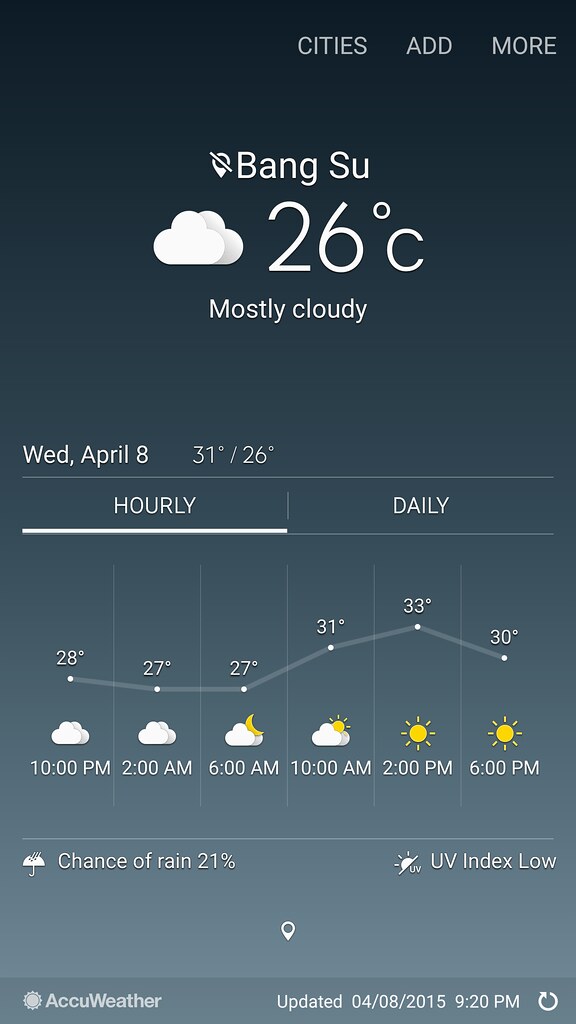The image depicts a weather app interface with a gray background and white and yellow icons. At the top of the screen, there are tabs labeled "Cities," "Add," and "More." The current selected city is "Bengsu." The main weather icon shows clouds and the temperature reads 26°C, indicating that it is mostly cloudy. Underneath the main temperature, additional details are provided: the day is Wednesday, April 8th, with a high of 31°C and a low of 26°C.

The interface features both an hourly and daily summary, with the hourly tab currently selected, highlighted by a white underline. The hourly forecast begins at 10 p.m., showing a temperature of 28°C with clouds. At 2 a.m. and 6 a.m., the temperature will be 27°C, accompanied by clouds. The 6 a.m. entry also includes a moon icon. At 10 a.m., the temperature rises to 31°C with partially sunny conditions. By 2 p.m., the temperature will peak at 33°C, and by 6 p.m., it will be 30°C and sunny.

Additional details indicate a 21% chance of rain and a low UV index. At the bottom of the screen, the app is credited to AccuWeather, with the last update timestamped 04-08-2015 at 9:20 p.m. A refresh symbol is located at the bottom corner of the interface.